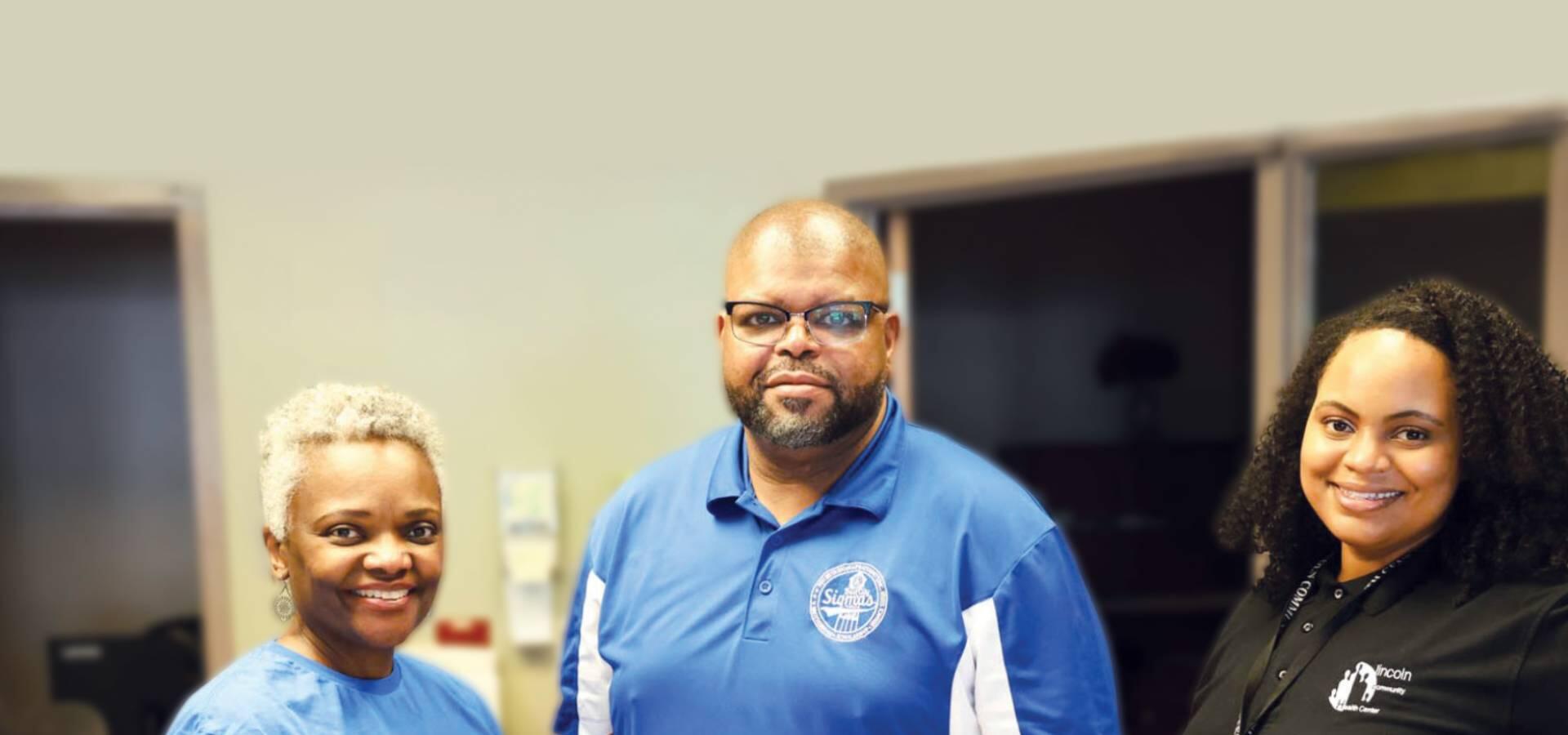This horizontally aligned, wide, but not very tall, indoor photograph features three smiling individuals. On the left is an African-American woman with short, blonde hair, wearing a blue shirt. The man in the middle has a bald head, short dark facial hair, and is dressed in a blue collared shirt with white print. He wears thick black-framed glasses. On the right stands another African-American woman with shoulder-length, thin braids. She is wearing a black shirt with white print. The blurred background reveals a room with light brown or very light gray walls, adorned with wooden trims around three doorways or windows. A doorway on the left leads to another room, while wood-framed doors or windows can be seen on the right. The wall has some kind of fixture, potentially a hand sanitizer dispenser. The overall atmosphere appears to be an office building.